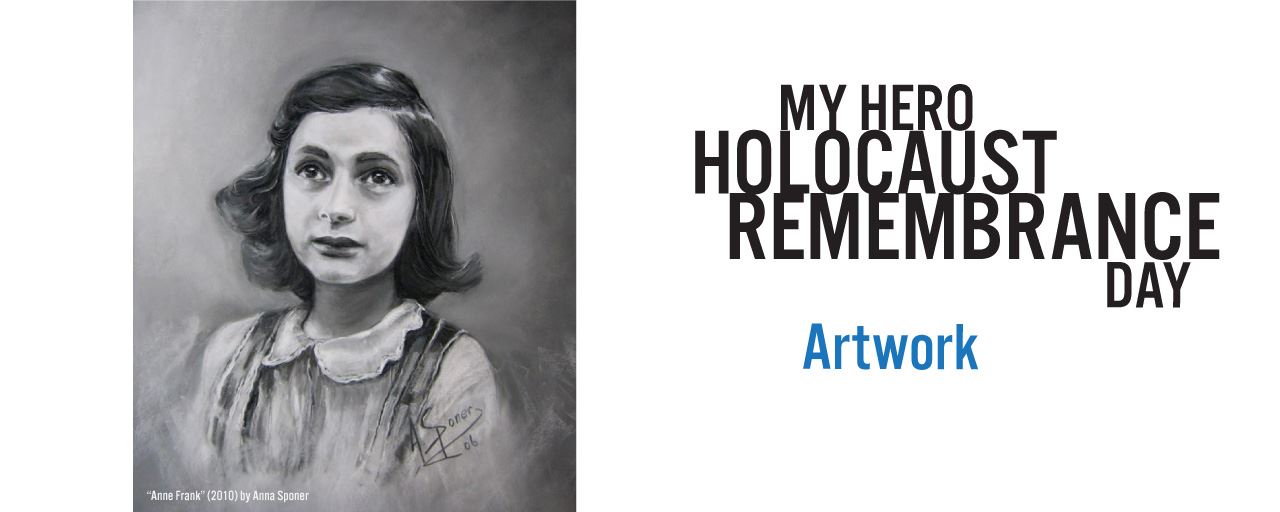The image is a black and white painting of Anne Frank, featuring her face and shoulders, set against a gray background that darkens on the right. Anne Frank, depicted with short, wavy, dark hair parted on the left, has a prominent nose and wears a dark-colored jumper with a white lace collar and white sleeves. She holds a solemn expression as she looks slightly upwards. The painting, signed by Anna Spencer in 2010 at the lower right, is titled "Anne Frank" in white letters beneath the image, accompanied by the artist’s name and date. To the right of the painting, the poster has a white background with bold black text near the top reading "My Hero Holocaust Remembrance Day" followed by "Artwork" in blue letters. This piece serves as a poignant tribute, capturing the enduring legacy of Anne Frank, whose diary chronicling her time in hiding during the Holocaust remains a significant historical document.